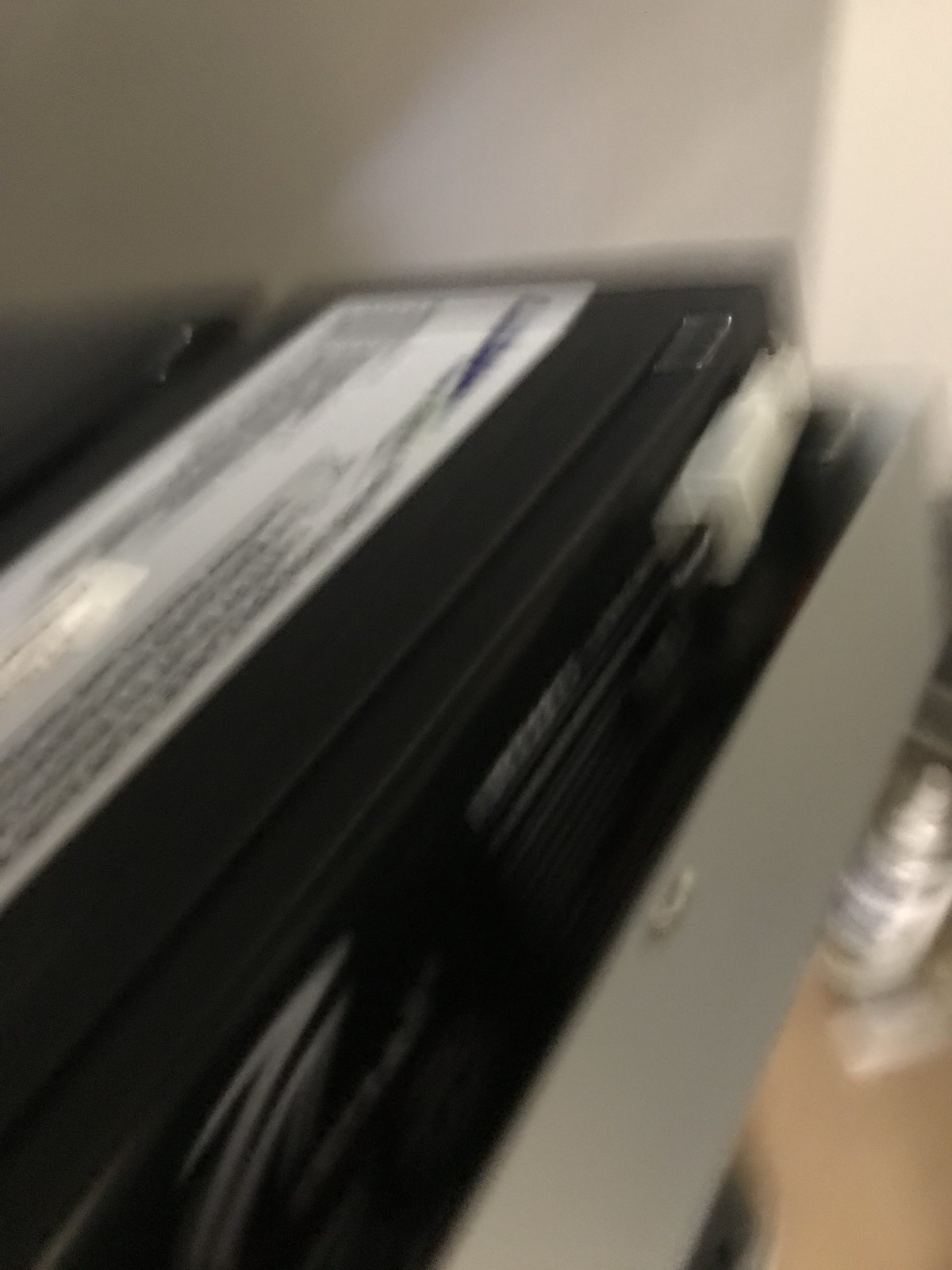This is a low-resolution, color photograph depicting a piece of office equipment, likely a copier or printer. The shot focuses on an open drawer within the machine, revealing a black surface on top. Inside the drawer, there is visible wiring and a small carriage assembly, suggesting the inner workings similar to that of a printer. The equipment is positioned against a neutral-colored wall, which is partly lit and casts a shadow from the machinery. The floor is partially shown, cluttered with miscellaneous objects, including what appears to be plastic packaging. A long label runs across the top of the equipment, although the lettering is unclear due to the poor photographic quality. Overall, the image gives the impression of a machine being actively repaired or inspected.